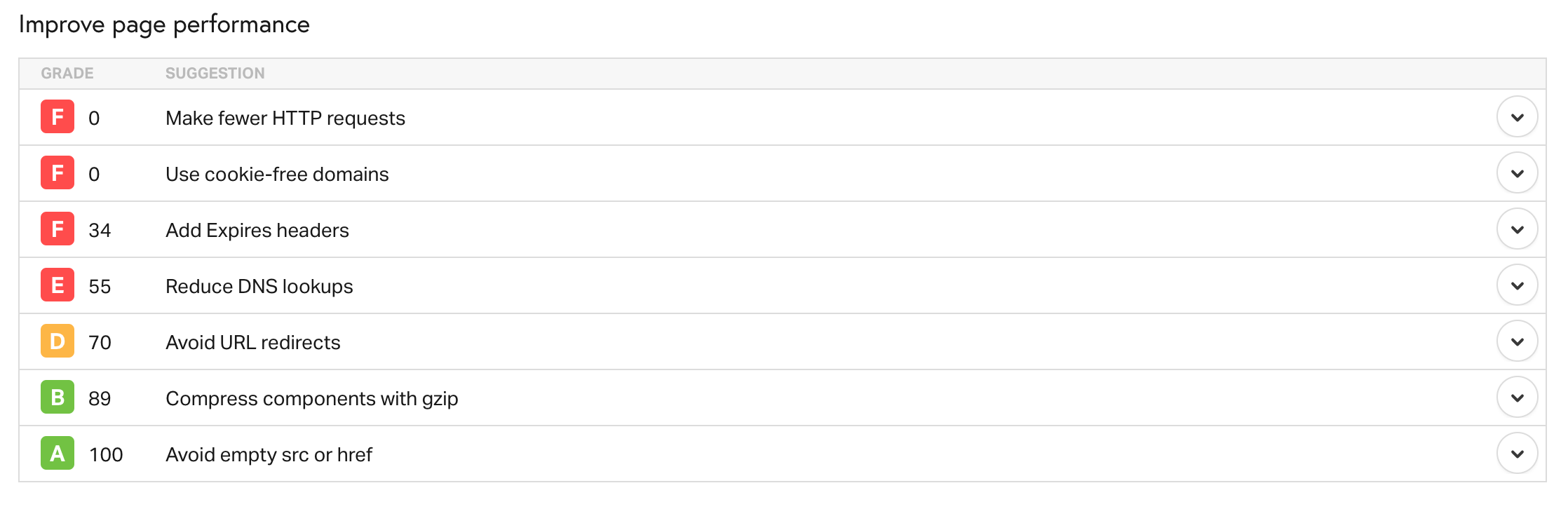**Caption:**

A detailed screen capture of a website performance evaluation tool is shown. At the top, the header in black font reads "Improved Page Performance". Below the header, a thin gray strip displays the labels "Grade" and "Suggestion". 

The main section of the image features a series of white boxes, each containing black font along with colored letters indicating grades. Each box also includes a white circle with a black pull-down arrow. 

1. The first box is marked "Grade F" with a red background and white "F", scoring zero. The suggestion is "Make fewer HTTP requests".
2. The second box, also graded "F" with a zero score, suggests "Use cookie-free domains".
3. The third box states "Grade F" with a score of 34, recommending "Add expires headers".
4. The fourth box carries a "Grade E" in a red box with a white "E" and a score of 55, suggesting "Reduce DNS lookups".
5. The fifth box is labeled "Grade D" in a gold box with a white "D", scoring 70, advising to "Avoid URL redirects".
6. The sixth box shows "Grade B" with a green background and a white "B", scoring 89, and suggests "Compress components with GZIP".
7. The final box features "Grade A" with a green background and white "A", scoring 100, with a suggestion to "Avoid empty SRC or HREF".

The image quality is excellent, with no blurring or pixelation, allowing the text and details to be clearly read. There are no other objects of interest in the capture.